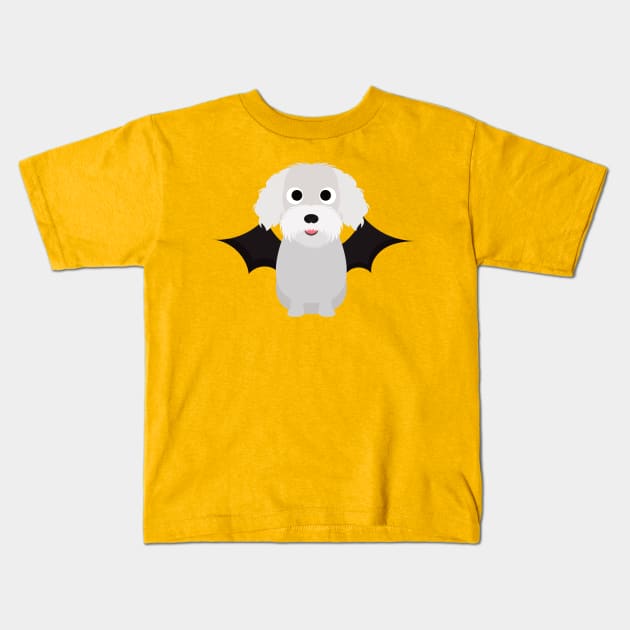This is a close-up picture of a small, short-sleeve child's yellow t-shirt, laid neatly on a white background with its arms spread flat. The shirt, a yellowish gold color, features a cartoon image of a gray dog prominently centered on the front. The dog, resembling a poodle, has white fluffy beard and ears, a black nose, and black eyes with large pupils. Its little open mouth reveals a bit of a red tongue. Attached to the adorable dog are stretched-out black bat wings, adding a whimsical touch to the shirt's design. Despite a few minor wrinkles, the t-shirt is presented in a tidy and clear manner, making all the details on the graphic easily visible.